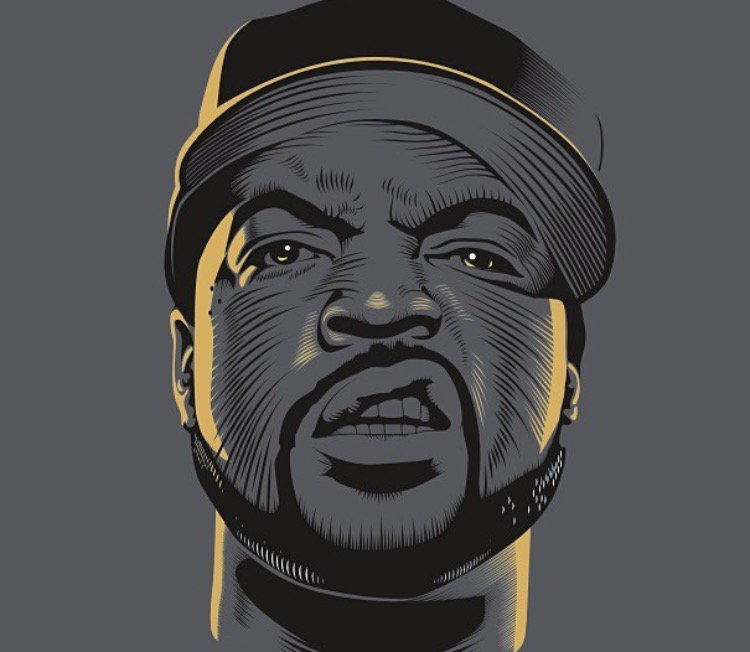This artistic illustration features Ice Cube, the renowned American rapper and actor known for his contributions to N.W.A, his solo rap career, and his roles in movies such as "21 Jump Street" and "Are We There Yet?" The drawing is executed in black ink on a dark gray background with subtle yellow highlights. Ice Cube is depicted from the neck up, facing the viewer with a distinctive sneer, displaying his slightly raised upper lip which reveals his teeth. He sports a black baseball cap tilted to the right, with a beard and mustache that fully encircle his mouth. His furrowed eyebrows intensify his expression, and the overall image is devoid of any text, artist attribution, other figures, animals, buildings, or mechanical objects, keeping the focus entirely on Ice Cube's iconic visage.